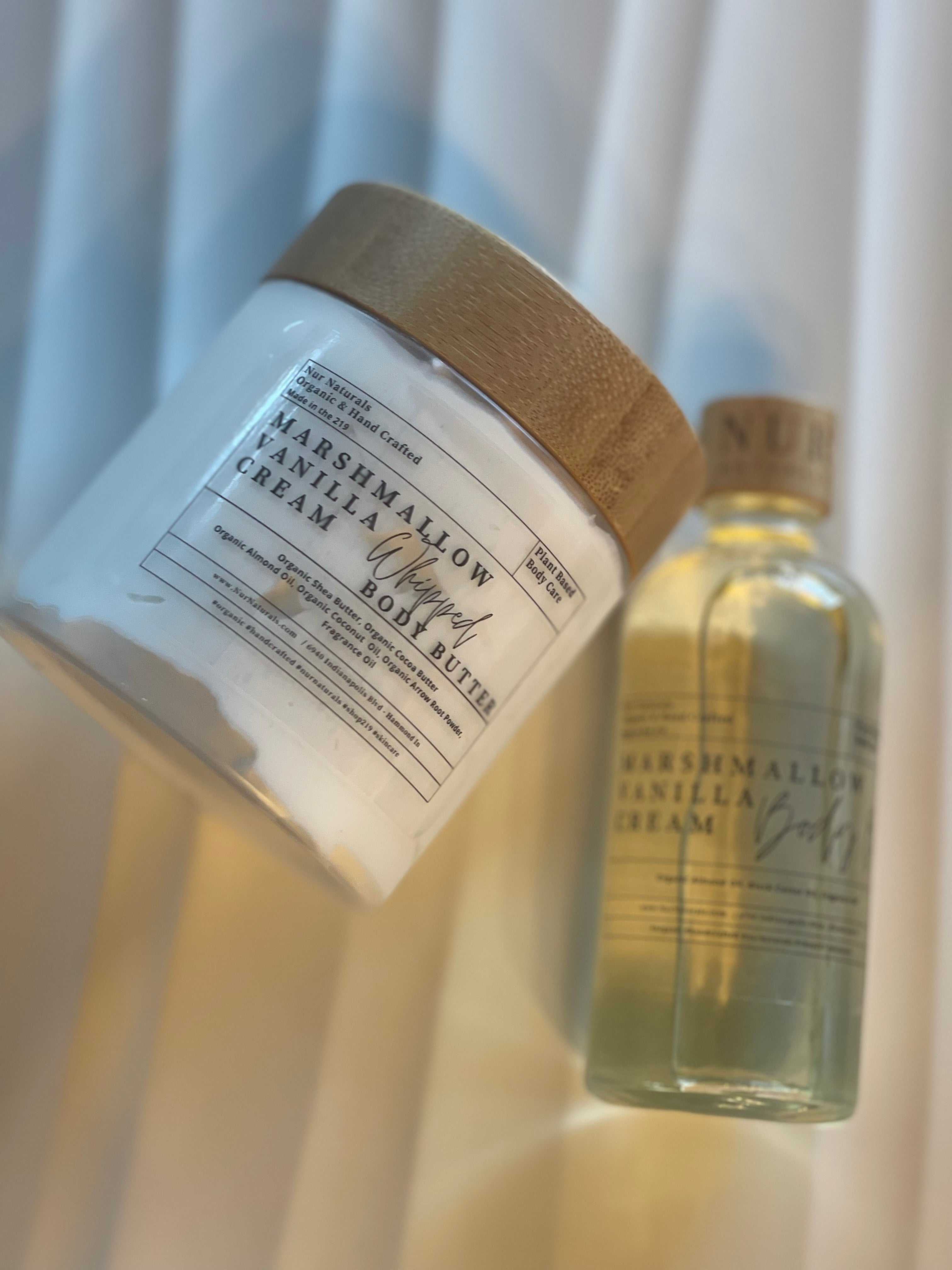The image is a close-up of two skin care products on a white textured surface. On the left is a small cylindrical jar made of clear glass, topped with a wooden circular cap. The jar's label in black text reads "Marshmallow Vanilla Cream Whipped Body Butter," with further small, illegible text underneath. The jar contains a thick, white cream. To the right, there is a slender glass bottle, also with a matching wooden cap. This bottle holds a light yellow, translucent liquid and bears the label "Marshmallow Vanilla Cream," although the remaining text is blurred and unreadable. Both products belong to the same fragrance line, suggesting they are complementary body care items designed for moisturizing the skin.